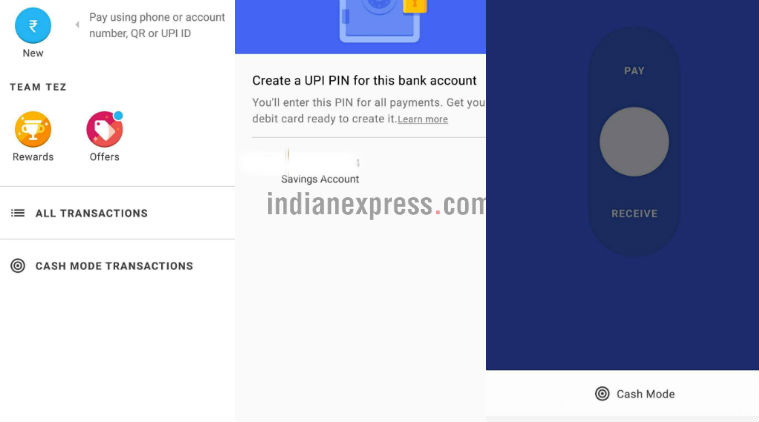The composite image showcases several adjacent computer screen snapshots, potentially of a mobile payment or banking application. The left section of the image features a screen with multiple payment options: "Pay using phone or account number," "QR or UPI ID," followed by the "Team Tez" branding. This section also highlights navigational links such as "Rewards and Offers," "All Transactions," and "Cash Mode Transactions."

The middle section displays content from "IndianExpress.com," suggesting a potential guide or user interface for creating a Unified Payments Interface (UPI) PIN for a bank account. It instructs the user to get their debit card ready to complete the PIN creation process, essential for enabling all payments.

The right section is slightly overlapped by another window, prominently showing a green slider button, labeled "Pay" and "Receive." This indicates a dual-functionality feature where the user can slide the button towards either option based on their requirement. Below this slider, the term "Cash Mode" is visible, hinting at a possible feature or transaction type within the application.

Overall, the composite image appears to provide a detailed guide on various functionalities of a financial application, from creating a UPI PIN to leveraging payment and transaction options.